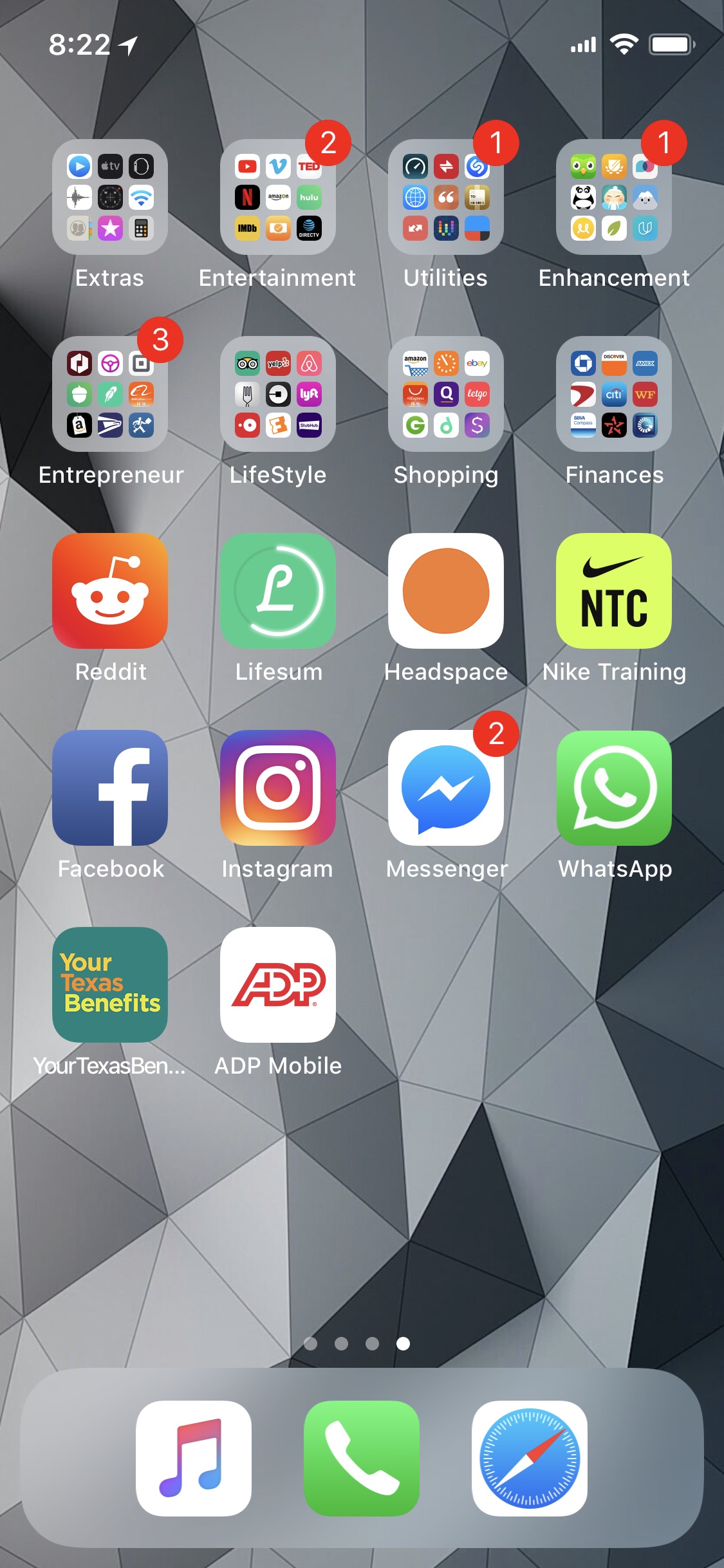Here is a cleaned-up and detailed caption for the image:

The image is a screenshot taken from a cell phone. In the upper left corner, the time displayed is 8:22. The top right corner shows the phone's battery icon, fully charged. 

The home screen is organized into several folders and apps. The first row includes folders named 'Extras,' 'Entertainment,' 'Utilities,' and 'Enhancement.' Each folder contains six app icons and features a red notification badge; 'Entertainment' shows a badge with the number 2, while 'Utilities' and 'Enhancement' both have the number 1.

In the second row, the folder 'Entrepreneur' displays a red badge with the number 3. This row also includes folders for 'Lifestyle,' 'Shopping,' and 'Finances.'

The third row features individual app icons: Reddit (orange with a white face icon), Lifesum (green), Headspace, and Nike Training.

The fourth row includes social media and communication apps: Facebook (blue with a white 'F'), Instagram, Messenger (with a red badge showing 2 notifications), and WhatsApp.

Beneath these rows, there is a green icon for text messaging and a white text box with 'ADP' in the center. The background of the home screen is patterned with gray diamonds.

Finally, on the bottom row, there are icons for Music, the Phone app (green with a white phone icon), and Safari (with a blue clock symbol).